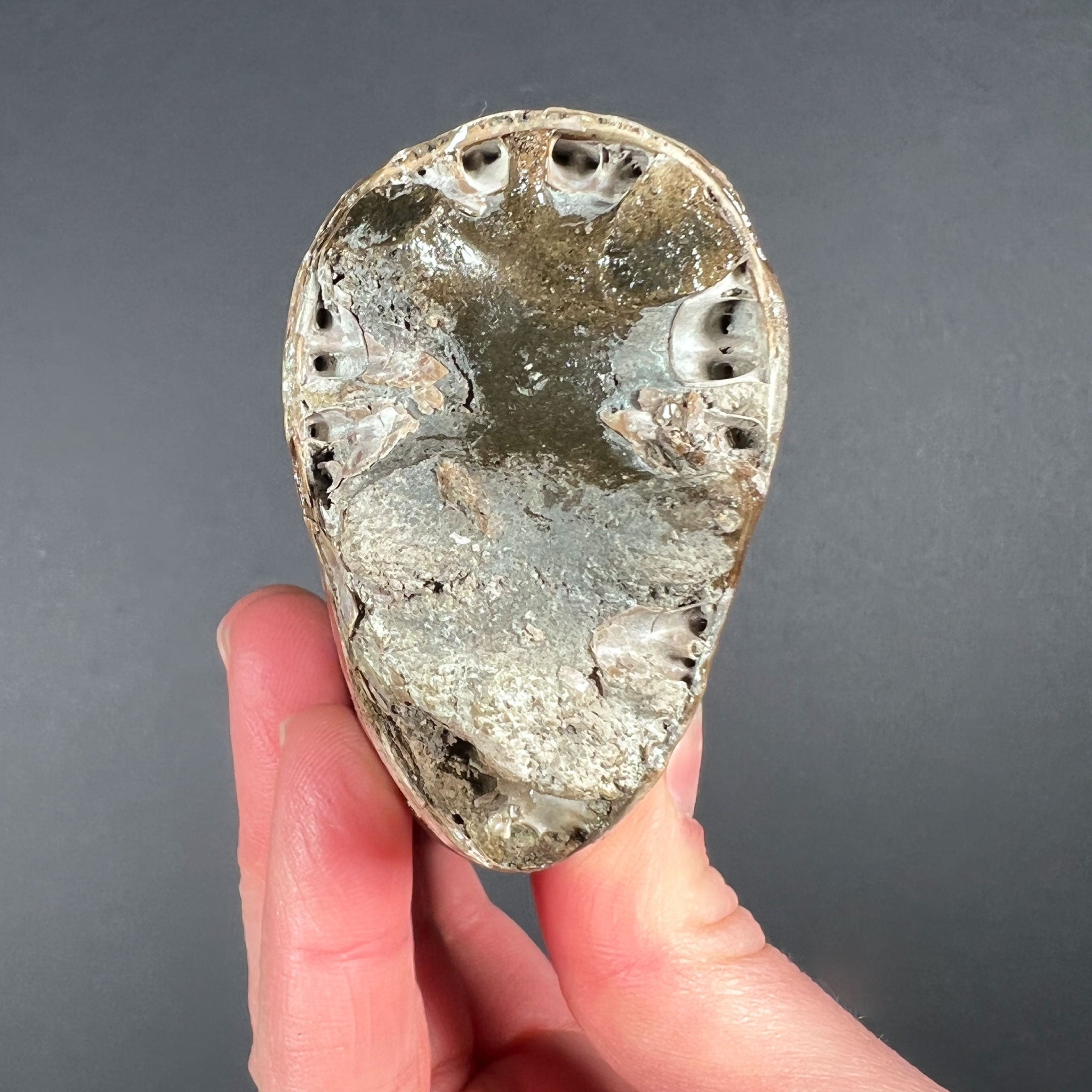In this close-up photograph, a human hand, likely the right one, holds a fossil-like object against a dark gray background. The object, resembling an oval or skull, features a wider top tapering to a narrower base. It has a bumpy gray texture with holes around what appears to be openings or the "head" area. The fossil displays portions of brown color interspersed with white spots, enhancing its intricate appearance. The person's hand, positioned around the object, reveals three or four fingers, with the thumb visible to the right and the other fingers, likely excluding the pinky, to the left of the object. The photograph captures the intricate details of the object's stone-like, possibly fossilized, texture, making the viewer focus on its unique formations.